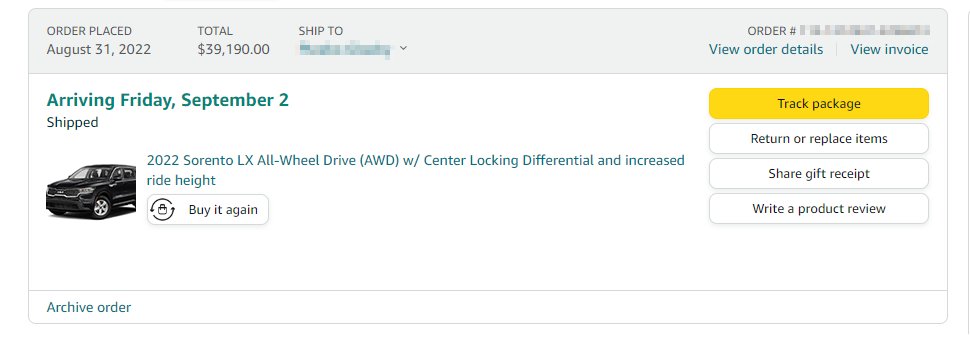Detailed Caption: 

The image features an order confirmation page for the purchase of a 2022 Sorento LX, an all-wheel-drive (AWD) black SUV. At the top of the page, it indicates that the order was placed on August 31, 2022, with a total price of $39,190. To the right, there is a section labeled "Ship To" where customers can view all the details and the invoice. The estimated arrival date is Friday, September 2, 2022. 

The vehicle description highlights its all-wheel-drive capability, featuring a center locking differential and increased ride height. On the left side of the image, a picture of the sleek black Sorento LX is displayed. To the right, several interactive buttons are visible, including "Buy It Again," a yellow "Track Package" button, and options to "Return or Replace Item," "Share," "Gift Receipt," or "Write a Product Review."